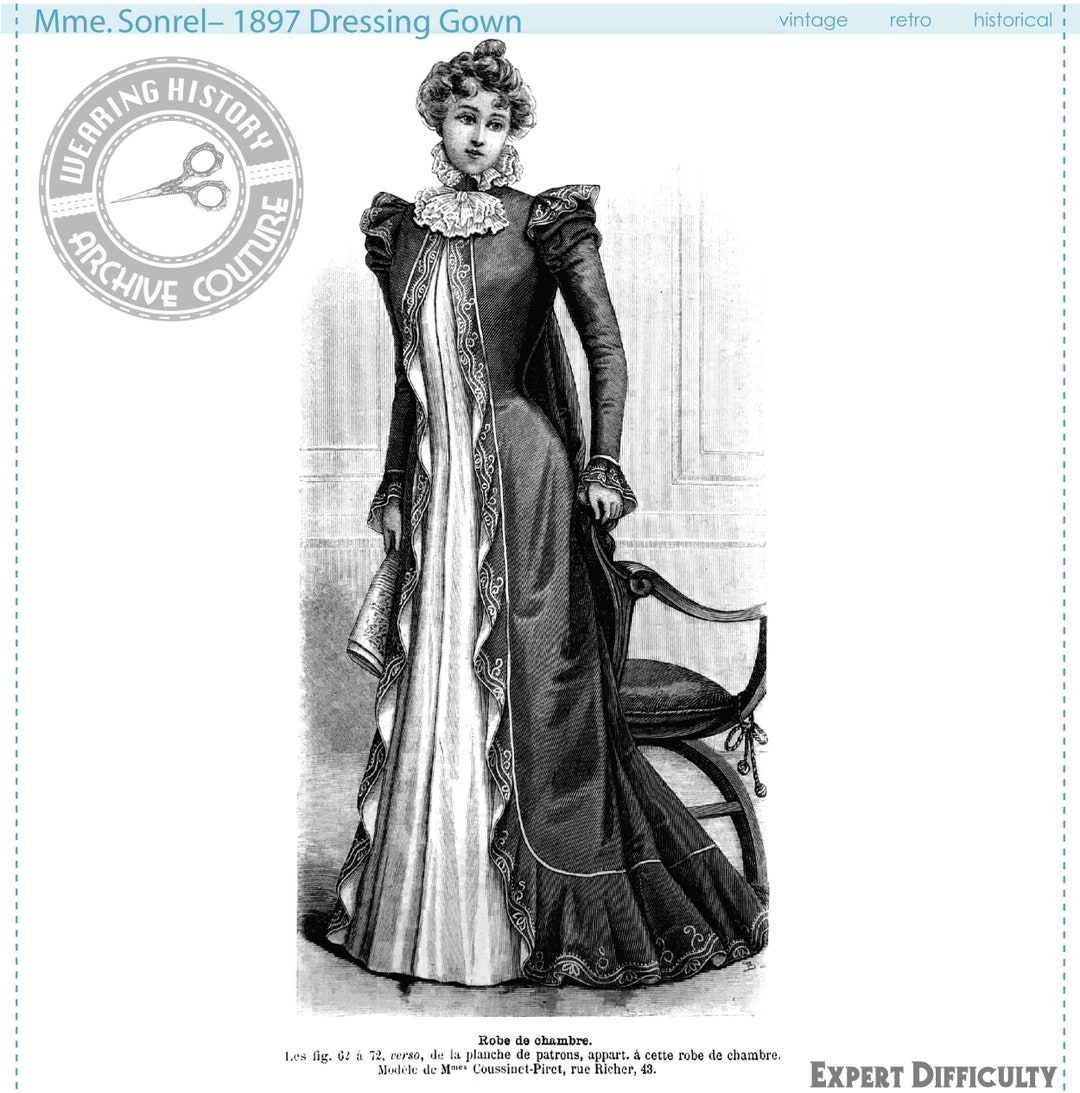The image is a highly detailed black and white drawing of a woman, presumably from the 1890s, specifically identified as Mademoiselle Sonrel. The top of the image features a caption that reads "MME Sonrel, 1897, Dressing Gown," along with the words "Vintage Retro Historical." To the top left, an oval logo compressed vertically reads "Wearing History, Archive, Couture," and features a pair of scissors in the center. The bottom of the image includes text in grey stating "Expert Difficulty" and a descriptive caption in French about the attire. The woman is dressed in an elaborate, floor-length gown with ruffles around her neck and chest. The gown opens in the middle to reveal a white interior. She has a high-laced collar and her hair is styled in an unusual updo with pointed buns. She stands with a neutral expression and her left arm rests on the back of a chair, which she appears to be leaning against for support. The background features a small wall, and there is additional text at the bottom to provide more context.